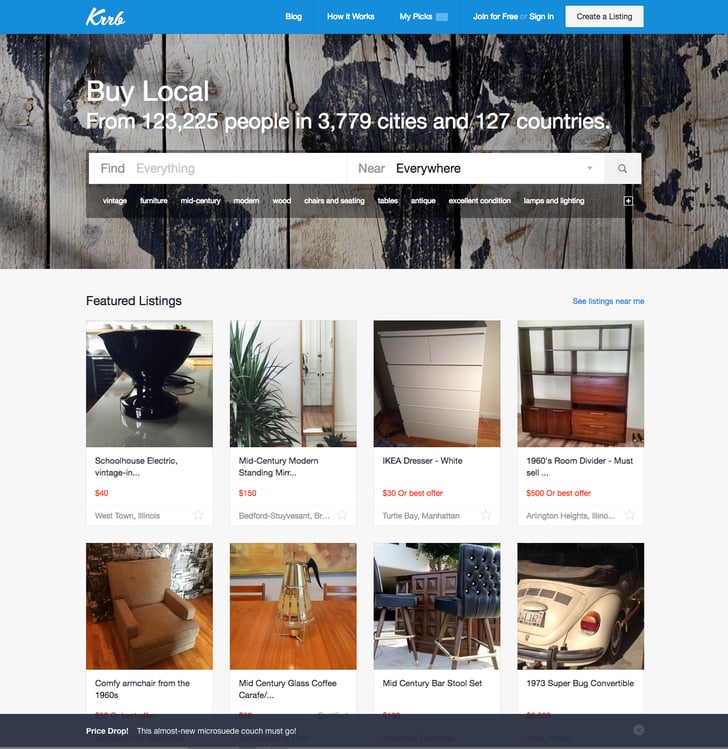This detailed caption describes a screenshot of the KRRB desktop application interface:

The screenshot features the homepage of KRRB, a company offering local buying and selling options. The top navigation bar includes options such as "Blog," "How It Works," "MyPix," "Join for Free," and "Sign In," all in white font floating against a vibrant blue background. A prominent white button labeled "Create a Listing" is also visible.

Below the navigation bar is an artistic world map rendered on a wooden texture. Overlaying the map is an invitation to "Buy local from 123,225 people in 3,779 cities and 127 countries," followed by a search bar with the placeholder text "Find everything near or everywhere." 

Further down, keywords such as "Vintage," "Furniture," "Mid-century," "Modern," "Wood," "Chairs and Seating," "Tables," "Antique," "Excellent Condition," "Lamps and Lighting" appear, with a plus sign indicating additional categories. 

The primary section showcases featured listings against a predominantly white background. Next to the listings, a blue hyperlink reads "See listings near me." The listings include images, descriptions, and prices; for instance, a "Schoolhouse Electric, Vintage Inn" priced at $40 located in Westtown, Illinois, and an "Ikea dresser, white, $30 or best offer" located in Turtle Bay, Manhattan.

At the bottom, set against a dark gray background, is a highlighted deal stating: "Price drop. This almost new micro suede couch must go."